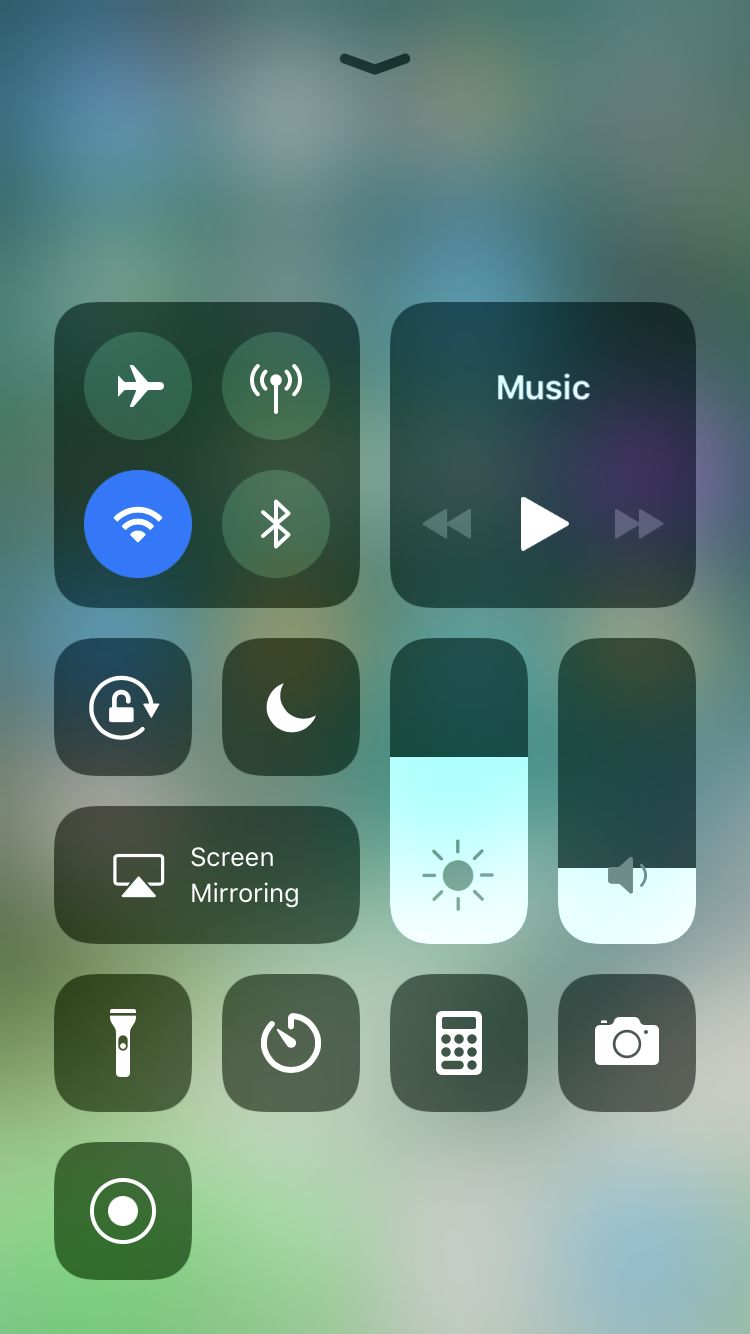The image depicts a control panel interface with various icons and symbols. At the top, there is a down arrow that appears slightly blurry due to the background. Below it, a circular icon contains symbols resembling a plane and radio signal, hinting at airplane mode and wireless connectivity functions. Surrounding this circle are indicators for full Wi-Fi signal, Bluetooth, and music controls flanked by left and right arrows and a play button.

A square labeled "Block Orientation" is also visible, possibly indicating a screen rotation lock feature. A half-moon icon below suggests a night mode or do not disturb function, while the right side shows a screen mirroring option. On the bottom left, there is a flashlight icon, and nearby, a circular icon—marked by a square symbol—may represent an app drawer or home screen.

Additional icons on the panel include a clock, a calculator, and a camera on the right. A brightness slider, illustrated with a sun symbol, lies next to a gray speaker icon. The overall background of the interface is very blurry, composed of muted shades of blue and green with a hint of purple in the bottom left corner. Various app icons are distributed towards the top of the image.